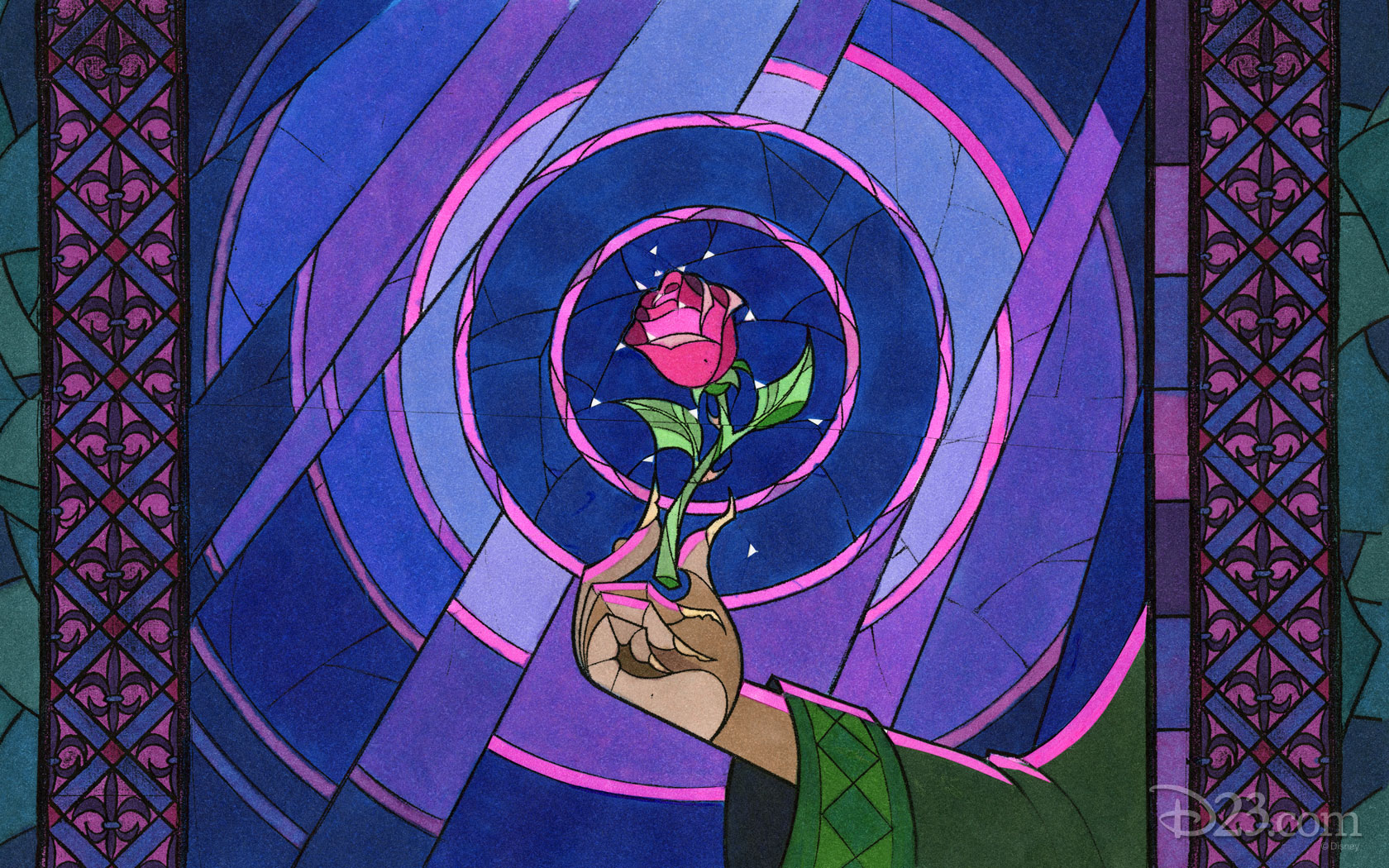This intricate cartoon stained glass artwork captures the essence of elegance and beauty with its detailed design. At its core, a vibrant pink rose with a single green stem and two lush leaves is delicately pinched between the thumb and forefinger of a person’s light tan-skinned hand. The person is adorned in a wide-sleeved green garment featuring decorative patterning around the wrist. Surrounding this central motif, a series of dark blue concentric circles spirals outward, although the circles become more disrupted and offset after the second round, suggesting a dynamic and fluid design. The background boasts a magnificent array of colors, including deep blues, pinks, purples, and lighter blues, creating a visually stunning yet harmonious effect. On either side of the image, ornamental and decorative vertical panels add to its sophistication. The bottom right corner is subtly marked with "d23.com," accompanied by the iconic Disney "D," hinting at the image's digital and branded artistry. Overall, this detailed stained glass image radiates brightness and color, achieving a perfect balance of complexity and elegance.